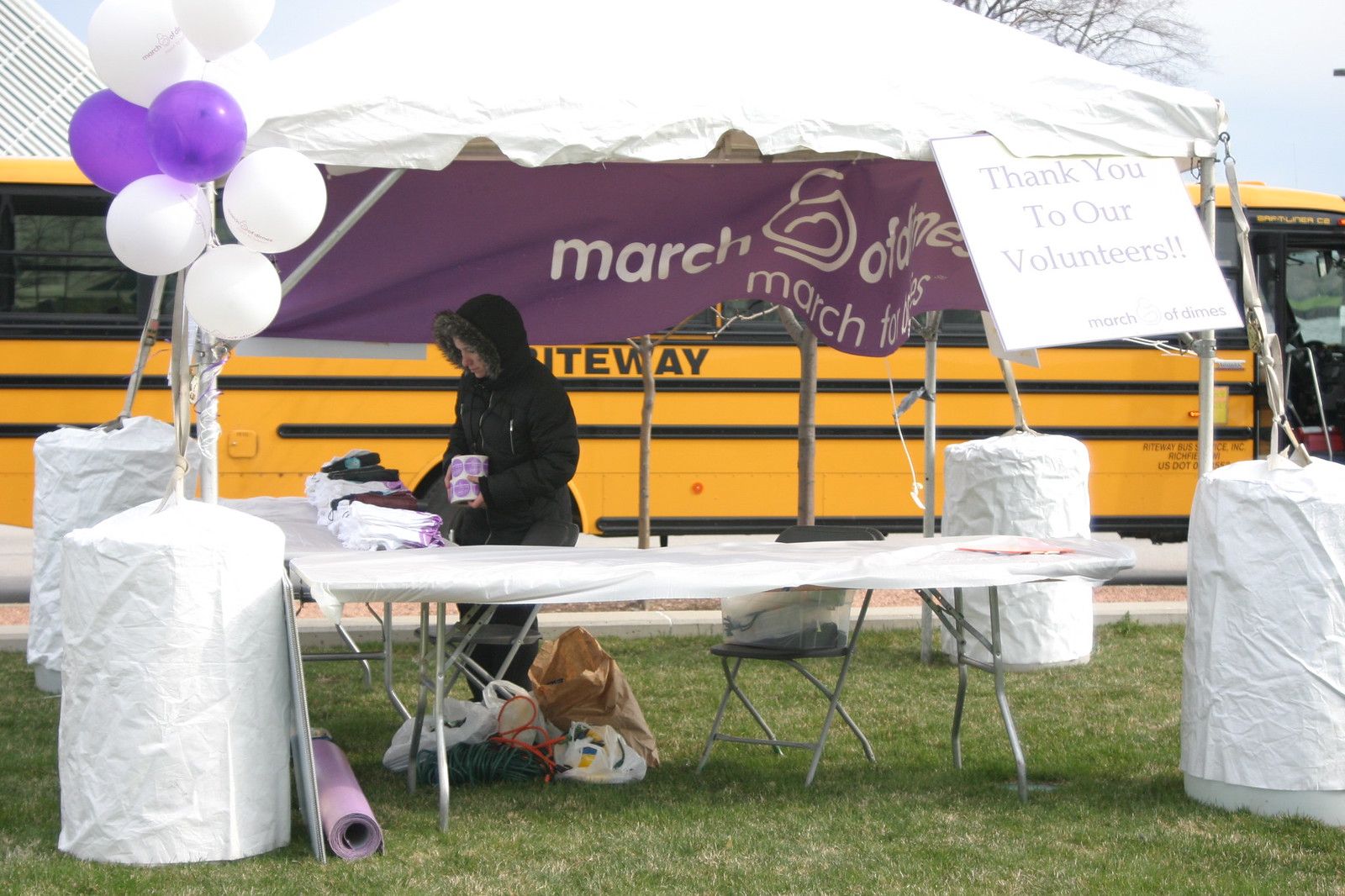A woman stands behind a portable table set up under a white event tent adorned with a purple banner that reads "March of Dimes, March for Babies.” The woman, dressed warmly in a black puffy jacket with a fur-lined hood pulled over her head, holds a container in her left hand, indicating the chilly weather. The table is covered with neatly folded clothes, which appear to be t-shirts, and underneath it, various bags and rolls of purple paper are visible. Tied to the table are white and purple balloons adding to the festive atmosphere.

The event takes place in a grassy area, and in the background, a yellow school bus can be seen parked under a bluish sky. On the left side of the tent, two white-covered cylindrical barrels have balloons attached to them, while similar barrels on the right side lack balloons but hold a sign expressing gratitude to the volunteers. A folding chair is also set up behind the table, adding to the scene's preparedness for the event activities.